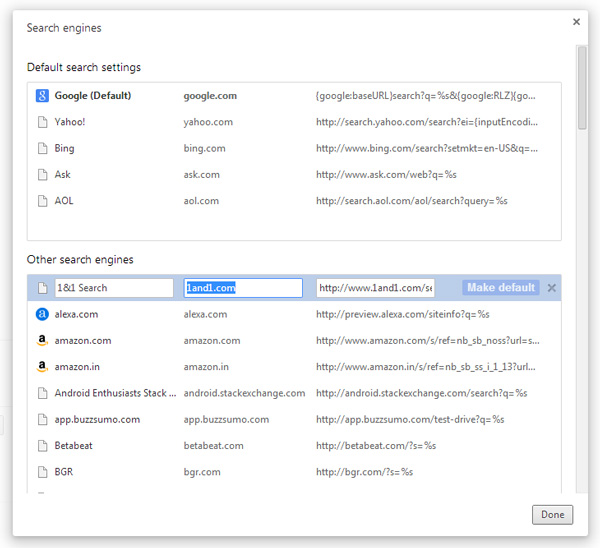Screenshot of a Search Engines Configuration Page:

The image is a detailed screenshot of a configuration page related to search engines. In the top left corner, there is a header that reads "Search Engines." The top right corner features a small black 'X', presumably for closing the window. Below the header, the page is divided into various sections for managing default search settings for five different search engines: Google, Yahoo, Bing, Ask, and AOL.

- Google is listed first and marked as the default search engine, with its corresponding URL displayed as google.com.
- Each of the other search engines, Yahoo, Bing, Ask, and AOL, also has their respective URLs listed.

Below this primary section is another list titled "Other Search Engines." This section includes text boxes with search engine information. For instance:
- The first text box contains "one-in-one search."
- The second box displays "one-in-one.com," which is highlighted.
- The final box features a web address alongside a blue button labeled "Make Default."

Furthermore, the page includes three columns: 
1. The first column shows the names of the search engines.
2. The second column presents simplified website addresses, such as alexa.com.
3. The third column displays extended URLs, example given is "http://preview.alexa.com."

Seven different search engines are listed under the "Other Search Engines" section.

At the very bottom right corner of the page, there is a "Done" button.